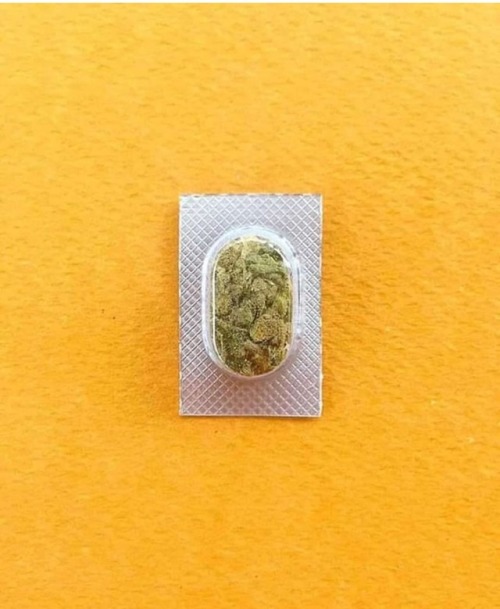The image displays a package of cannabis flowers resting on a textured mustard-yellow surface. The cannabis flowers are housed within a clear, oval plastic cover, which is wrapped in a silver cardboard package adorned with a lead pattern. The green cannabis flowers inside show signs of mold. The entire package, including the clear plastic and silver cardboard, sits on top of what appears to be a white napkin, adding a subtle contrast to the mustard-yellow background. The plastic cover is oval-shaped, and the flowers inside are distinctly visible due to the see-through nature of the cover. The textured yellow surface beneath adds dimension to the overall presentation of the package.